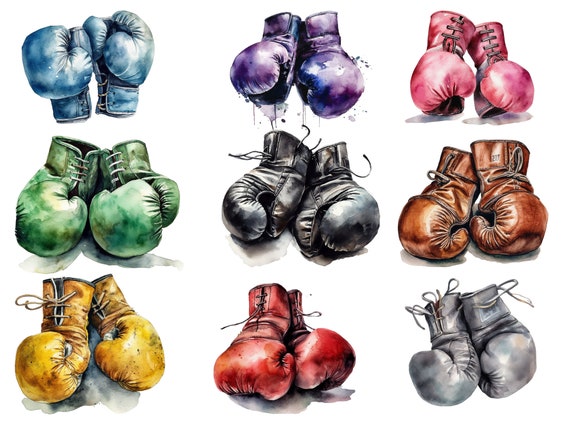The image displays nine pairs of painted boxing gloves, arranged in a 3x3 grid on a white background. Each pair of gloves is a different color and in varying positions. The colors, from top left to bottom right, are blue (pointing up), purple (pointing down), pink (pointing down), green (pointing down), black (pointing down), brown (pointing down), yellow (pointing down), red (pointing down), and gray (pointing down). Each glove pair is laced up with matching colored ties around the wrists, and some gloves feature subtle watercolor shadowing beneath them. The gloves are artistically rendered to appear as if they are floating, with no physical borders or additional context.